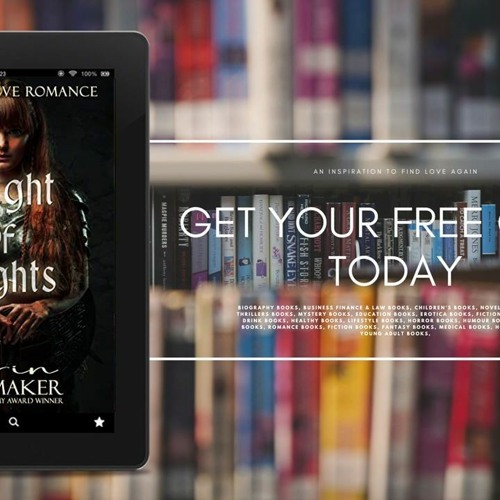This photograph appears to be an advertisement prominently featuring a Kindle e-reader on the left side of a square image. Only about half of the Kindle is visible, showcasing a black border. On the top left corner of the Kindle's screen, the battery percentage and related status icons are displayed in white. The Kindle screen displays a book cover, with the word "romance" clearly readable, although the rest of the text is not discernible. 

The background of the entire image consists of shelves filled with books, with most of them blurred to draw focus. Only a small band of books in the center remains clear. Over this clear section, in bold white block capital letters, is the promotional text "GET YOUR FREE TODAY." This text is framed by a white horizontal line above and below it. Below the word "TODAY," there is some additional smaller white text, which is too small to be read clearly.

This detailed composition underscores an enticing offer and the captivating allure of romance novels available on the Kindle.